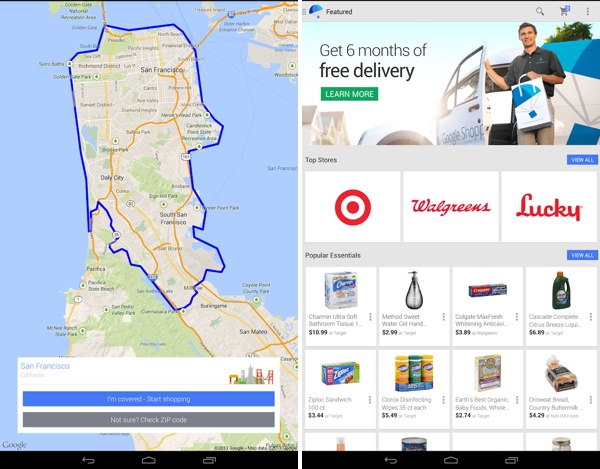This image illustrates the delivery area available in San Francisco along with a list of participating stores for local deliveries. On the left side, a map of San Francisco is prominently displayed, bounded by a blue border that delineates the delivery zone. The map includes labels for various nearby locations such as Daly City, Brisbane, South San Francisco, and Pacifica, though the text is slightly blurry. Areas outside the blue-bordered delivery zone are also visible on the map.

To the right side of the image, there is a photograph of a man standing beside an open vehicle door. He is holding a shopping bag characterized by a white background and a blue umbrella logo. The side of the vehicle partially reads "Google shop." Just above the car, there's a promotional message stating "Get six months of free delivery."

Below this image, a list of top stores is provided, featuring logos from Target, Walgreens, and Lucky. Underneath these logos, the caption "popular essentials" is displayed above images of eight household items, including bath tissue, Ziploc sandwich bags, and Cascade. Each product is accompanied by its name, price, and the store from which it can be purchased.